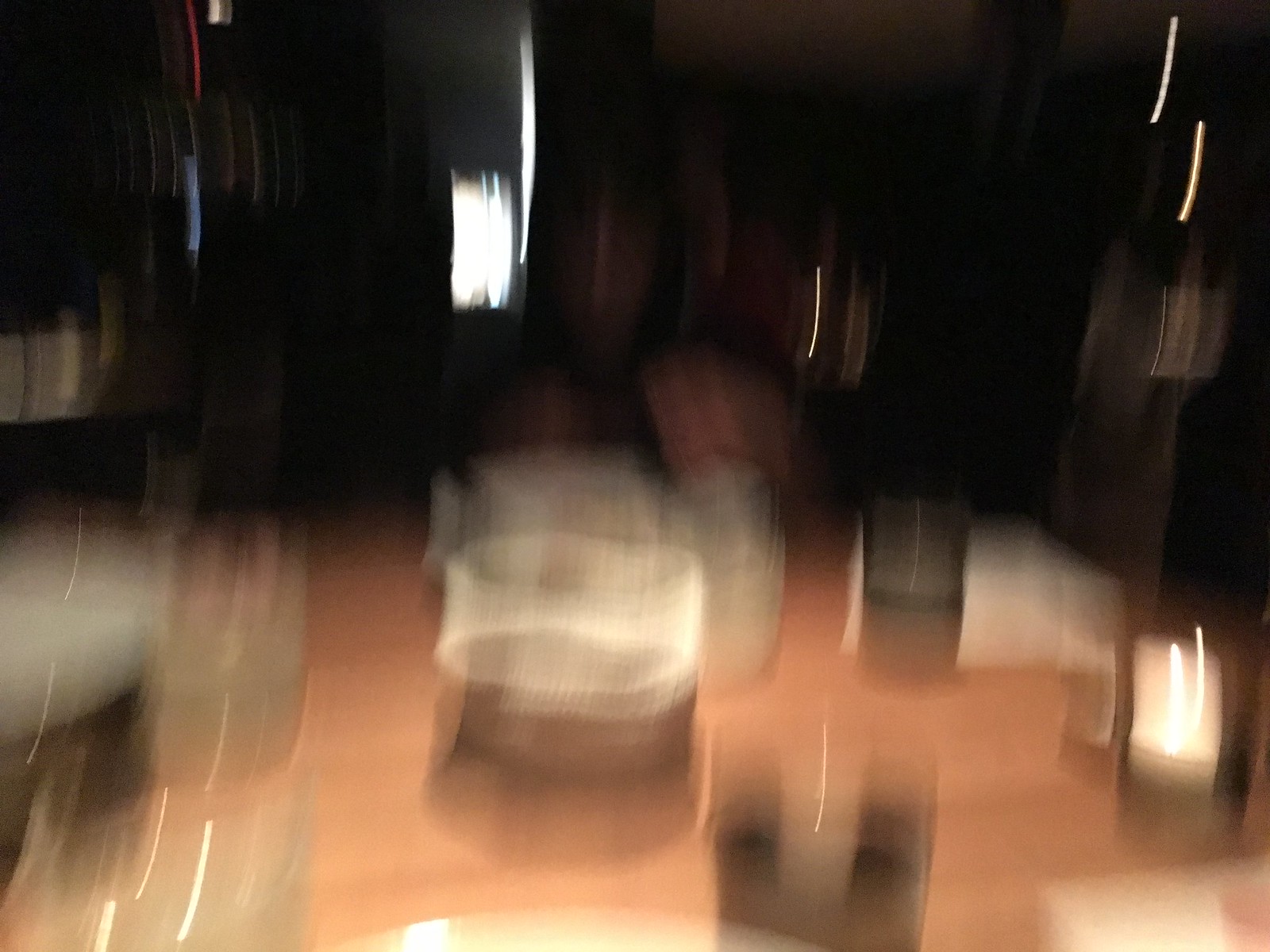The image depicts a very blurry scene with a dark black background illuminated by flashes of light, particularly towards the top left corner. Below, there is a light brown hardwood floor. In the foreground, several cups or glasses rest on a round, possibly wooden countertop or table. The glasses appear to be a mix of clear and dark, smoky-like materials. One glass on the right side seems to be either lit or reflecting a nearby light source. Amidst the unclear image, there might be a person seated in the background, though it is indistinct. To the left, another counter or piece of equipment is faintly visible, and a light source, possibly from a window, casts some illumination in the background. The overall scene is ambiguous, potentially depicting either a casual setting with drinks being enjoyed or a display of candles.